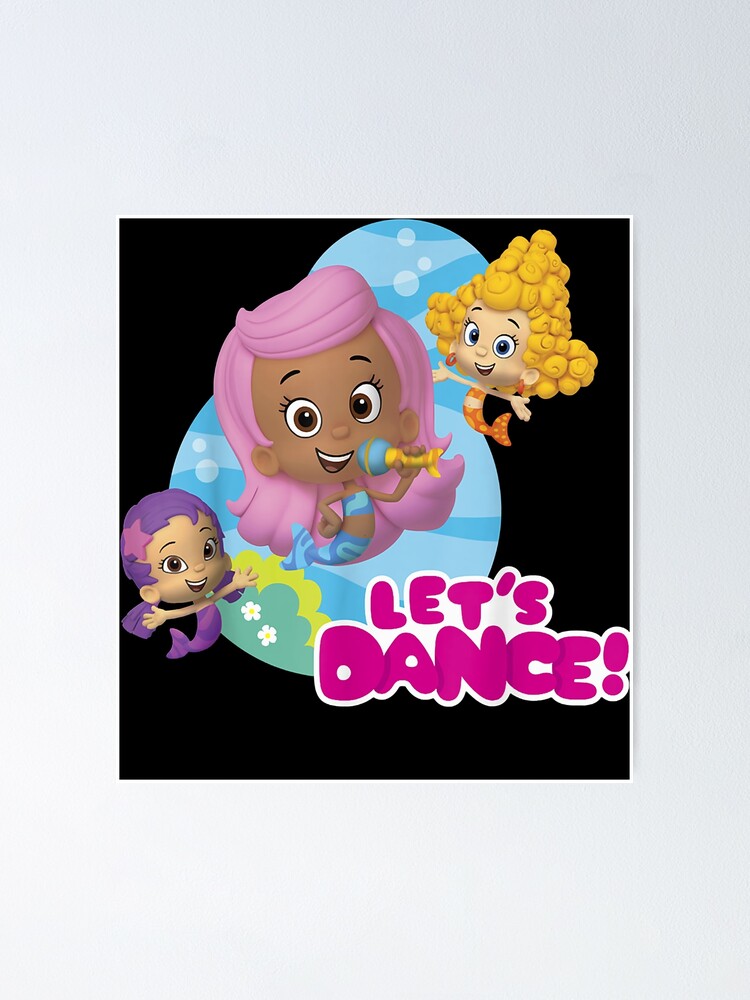The image is a colorful cover for a children's show featuring three animated mermaid characters set against a dynamic water-themed backdrop. The central background is black, while the surrounding area has light blue and deeper blue ocean waves, bubbles, and ocean plants, creating an underwater scene. At the bottom right corner, the phrase "Let's Dance!" is prominently displayed in large, fluffy, dark pink letters with a white shadow.

The three cartoon mermaids are each distinct in appearance. The girl in the middle has darker skin and pastel pink hair, wearing a blue striped outfit and holding a blue microphone with a fishtail-shaped detail, suggesting she is singing. To her left, a darker-skinned girl with purple hair is dressed in a purple bikini top. On the upper right, a white girl with bubbly blonde hair is sporting an orange polka-dotted outfit with matching orange earrings. All three characters are floating, emphasizing their mermaid forms and creating a lively, musical, and vibrant scene perfect for a children's program.